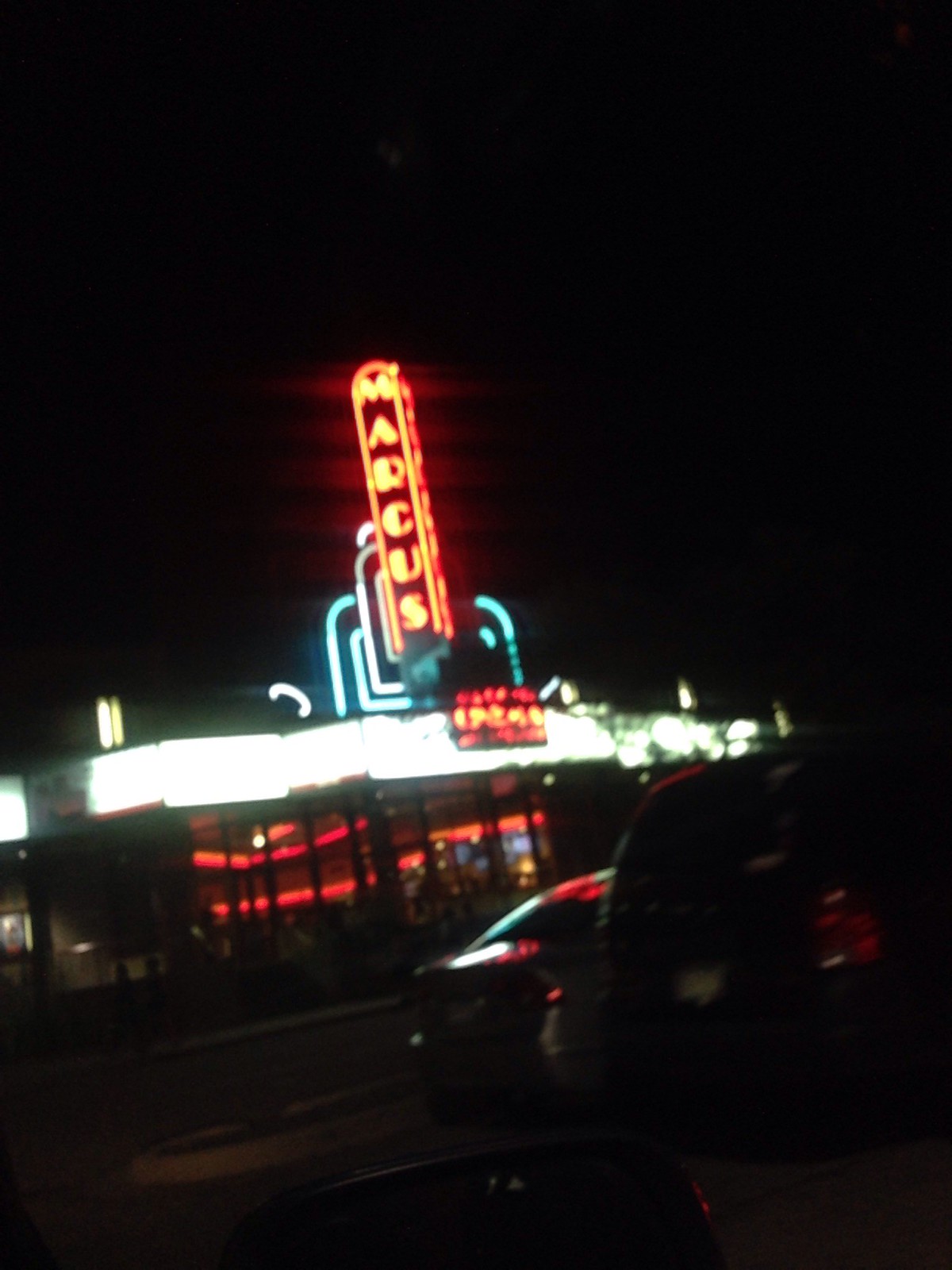The photograph captures a nighttime scene viewed from the passenger side of a car, with the window partially rolled down. Despite its blurriness, the bustling atmosphere outside comes through. In the background, a modern restaurant named "Mad Kiss" stands out, adorned with bright, colorful lights that illuminate the surroundings. Through the haze, the restaurant's red interior lights cast a warm glow, hinting at a lively, crowded establishment. The scene also includes other vehicles, notably a van and a sedan, parked nearby, which further enhances the sense of an active, vibrant night.